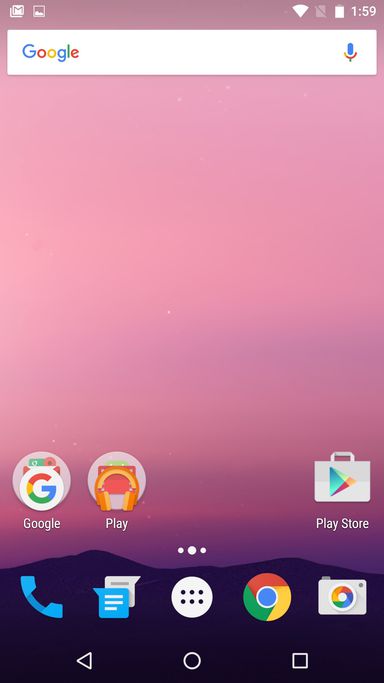The screenshot showcases the home screen of a smartphone featuring a visually appealing background. The top portion of the screen displays a light lavender sky that gradually darkens into a rich purple hue at the bottom, resembling a serene mountain range at dusk. 

At the top right corner, the time is clearly visible in white font, reading 1:59. Alongside the time, there are icons indicating battery life and Wi-Fi connectivity. On the left side of the screen, the Gmail icon is prominently displayed.

Just below the top border, there's a Google search box, showing the company’s logo styled with its customary vibrant colors: a blue "G," red "O," yellow "O," blue lowercase "g," green "L," and a red "E." To the right of the search box is a blue microphone icon.

At the bottom of the home screen, three key apps are aligned: the Google app, one labeled "Play," and the Google Play Store. The Play Store icon is distinctive, portrayed as a white suitcase containing a prism in Google’s signature colors.

Further down, four essential icons are situated: the phone app, text messages, Google Chrome, and what appears to be Google Documents. At the extreme bottom, navigation icons are visible, including an outlined circle in the center, a triangle pointing left on the left side, and a square on the right side, facilitating easy access and navigation.